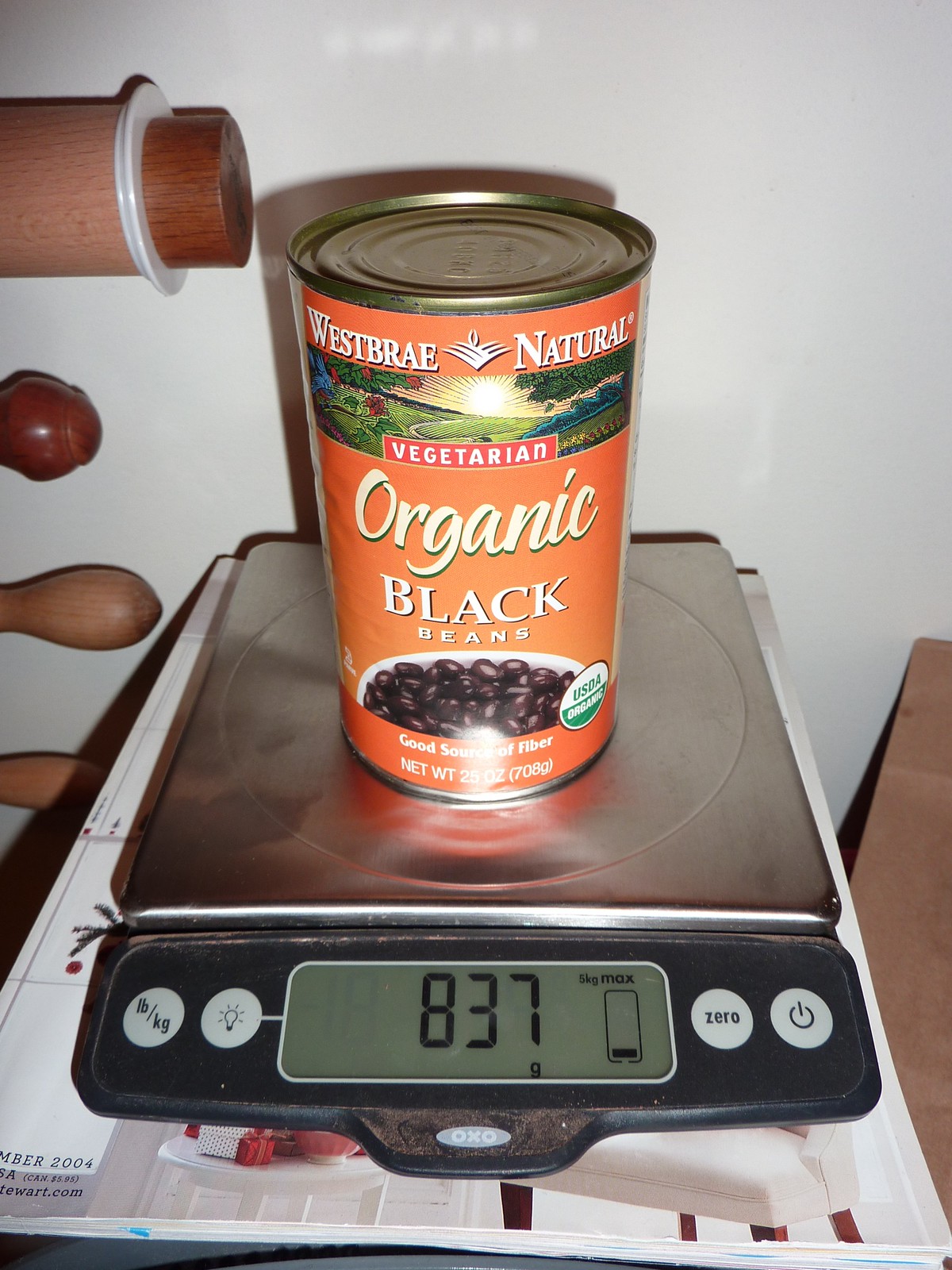This image, taken in a kitchen, showcases a can of West Bray Natural Vegetarian Organic Black Beans on a silver and black digital kitchen scale with a black face. The scale, which reads "837 grams," displays circular buttons including LB/KG, a light bulb icon, a zero button, and a power button, with a small spherical button labeled "OXO" underneath the screen. The can, with an orange label, features a sunrise illustration over green fields and trees, and an image of black beans in a white bowl, highlighting that it is a good source of fiber with a net weight of 25 ounces (708 grams). To the left of the scene, wooden kitchen tools are hanging on a white wall, and the scale is positioned on top of a magazine. The detailed label includes a USDA Organic emblem, emphasizing the beans' organic nature.